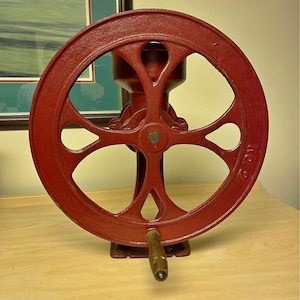In the image, we see a striking red antique machinery, possibly a coffee grinder or mill, resting on a light wood-colored table. The circular device, primarily composed of metal and painted red, features a translucent midsection, allowing a view of its inner mechanics. Surrounding the center are other circular components, and a golden brass handle is affixed at the bottom, designed to rotate the mill or wheel. This handle can be cranked clockwise or counterclockwise, suggesting the mechanism is used for turning or adjusting something significant, potentially a valve. The setting appears to be a museum or exhibit, indicated by the careful display on the wooden platform. In the background, part of a painting is visible on the white wall, along with the faint reflection of the photographer in the picture frame.